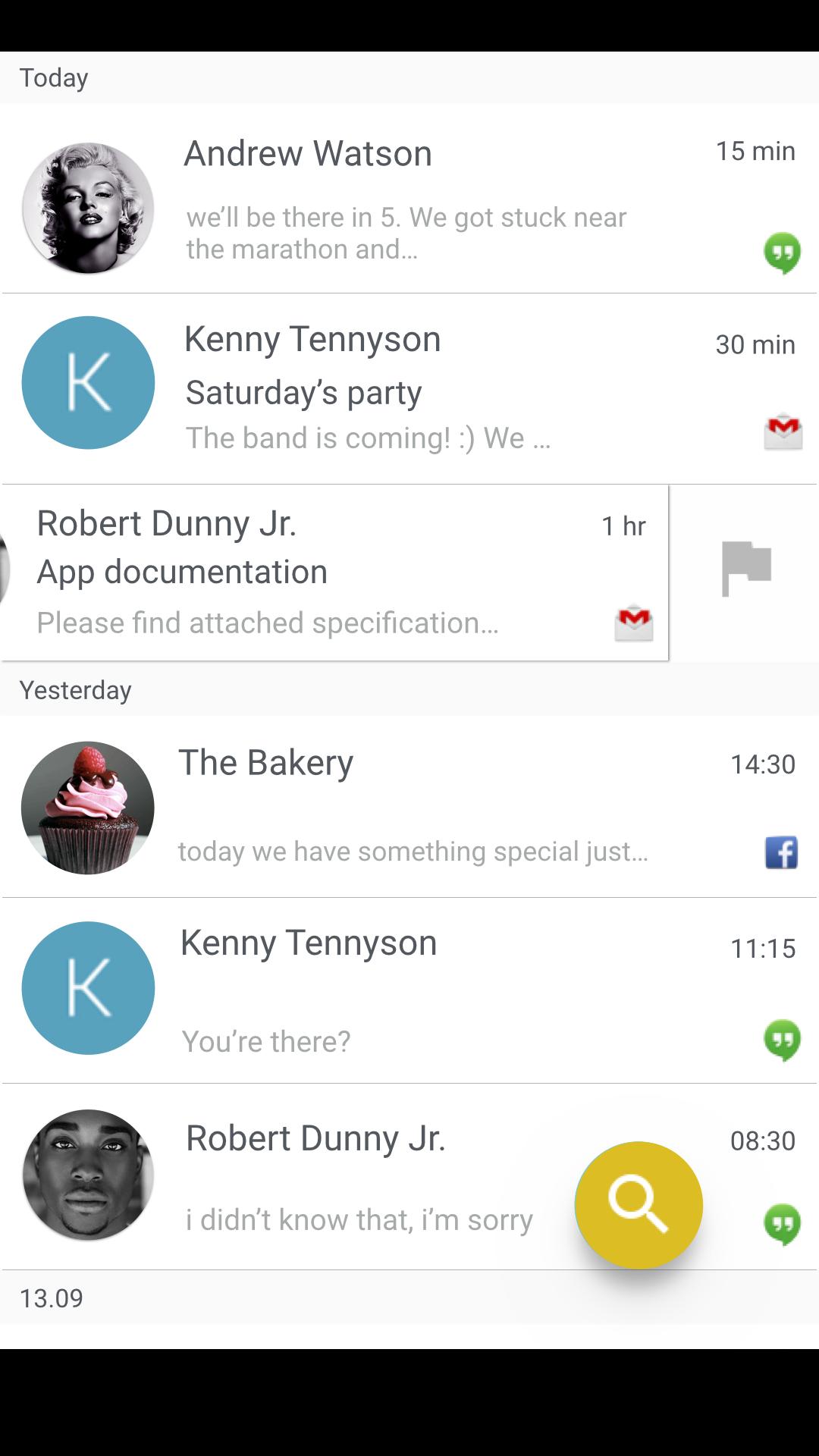Here is a cleaned-up and detailed caption for the image you described:

---

**Screenshot of Various User Comments** 

The image captures a series of comments with timestamps, arranged in chronological order. At the top, it states "Today." The first comment is from Andrew Watson, whose profile picture is an image of Marilyn Monroe. Andrew states, "We'll be there in five, we got stuck near the marathon," indicating 15 minutes ago.

Below that, a comment from Kenny Tennyson is displayed. Kenny's profile picture features a blue circle with a white "K." He says, "Saturday's party, the band is coming :)," showing it was posted 30 minutes ago.

The next comment, from Robert Dunney Jr., reads, "App documentation: Please find the attached specification," posted one hour ago.

Following that, a section labeled "Yesterday" appears. The bakery, represented by a profile picture of a chocolate cupcake with pink frosting topped with a raspberry, posted, "Today we have something special," at 14:30 (2:30 PM).

Further down, another comment from Kenny Tennyson asks, "You there?" timestamped at 11:15. 

The final comment in the screenshot is from Robert Dunney Jr., expressing, "I didn't know that, I'm sorry," seen next to a profile picture of a golden circle with a white magnifying glass (search button), posted at 08:30.

---

This caption provides a clear and detailed summary of the content in the image.